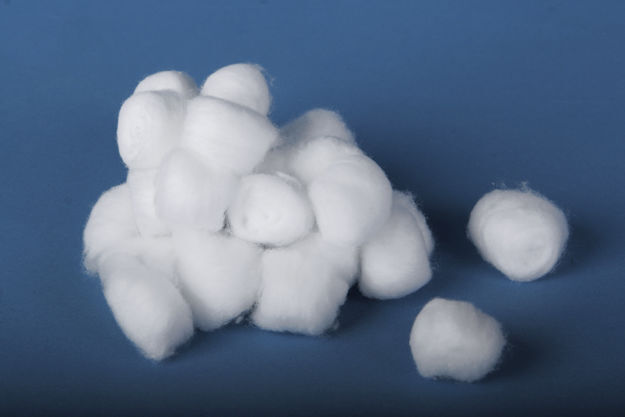In this detailed image, set against a gradient navy blue background that transitions from a darker shade at the bottom to a lighter shade at the top, there is a central focus on a strategically arranged pile of white cotton balls positioned towards the left-hand side. The artistic arrangement resembles that of a car, with a solid base layer composed of approximately 15 to 20 cotton balls, a middle layer with about 9 to 10 cotton balls, and a top layer capped with 4 or 5 balls. In the lower right-hand corner, two individual cotton balls sit separately, adding to the composition's dynamic balance. This central pile and the individual balls cast subtle shadows on the cobalt blue backdrop, creating a sense of depth and three-dimensional form. The overall scene evokes the impression of a child's creative school art project, showcasing both the imagination involved in constructing with cotton balls and the interplay of light and shadow on the richly colored background.